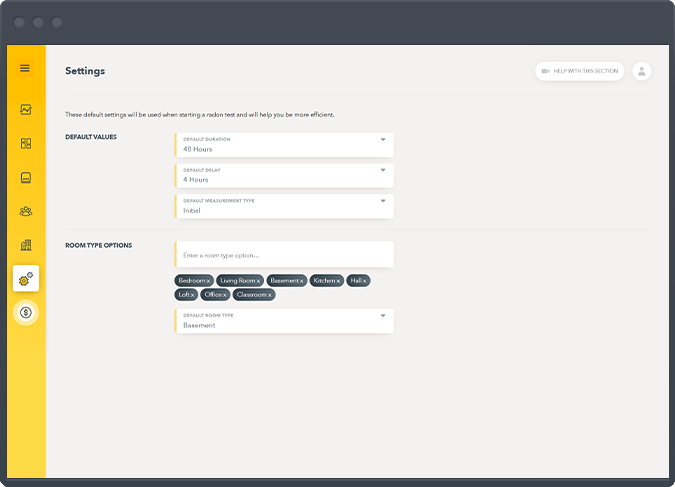The image showcases a screenshot of a settings panel, presented as a mock-up within a browser-like window. The window has a sleek, dark gray flat design, with three dots located in the upper left corner, hinting that it might be intended for a Mac interface. 

On the left side of the panel, there is a vertical menu styled in a flat yellow background. This menu includes various icons arranged vertically from top to bottom: a hamburger menu icon, a graph, an eye icon next to an inverted eye icon, a square with rounded corners containing an underscore, three icons representing people (one centered and two behind), two building icons, a gear icon within a white square, and finally, a dollar sign enclosed in a white circle.

In the main section of the settings panel, text instructions indicate that "These default settings will be used when starting a Radon test, and will help you be more efficient." There are several specific settings listed, including:

- **Default values**
- **Default duration**: 48 hours
- **Default delay**: 4 hours
- **Default measurement type**: Initial
- **Room type options**: Users are prompted to enter room type options. Predefined tags available include bedroom, living room, basement, kitchen, hall, loft, office, and classroom. Each tag has an 'X' that can be clicked to remove it.

Below these tags, there is another input field labeled "Default room type," which is currently set to "basement."

In the upper right corner of the main settings area, there is an icon resembling a video camera with the text "Help with this section" next to it, as well as a simple profile icon.

This detailed layout of the settings panel provides a clear and comprehensive understanding of the configurable options available for setting up a Radon test.